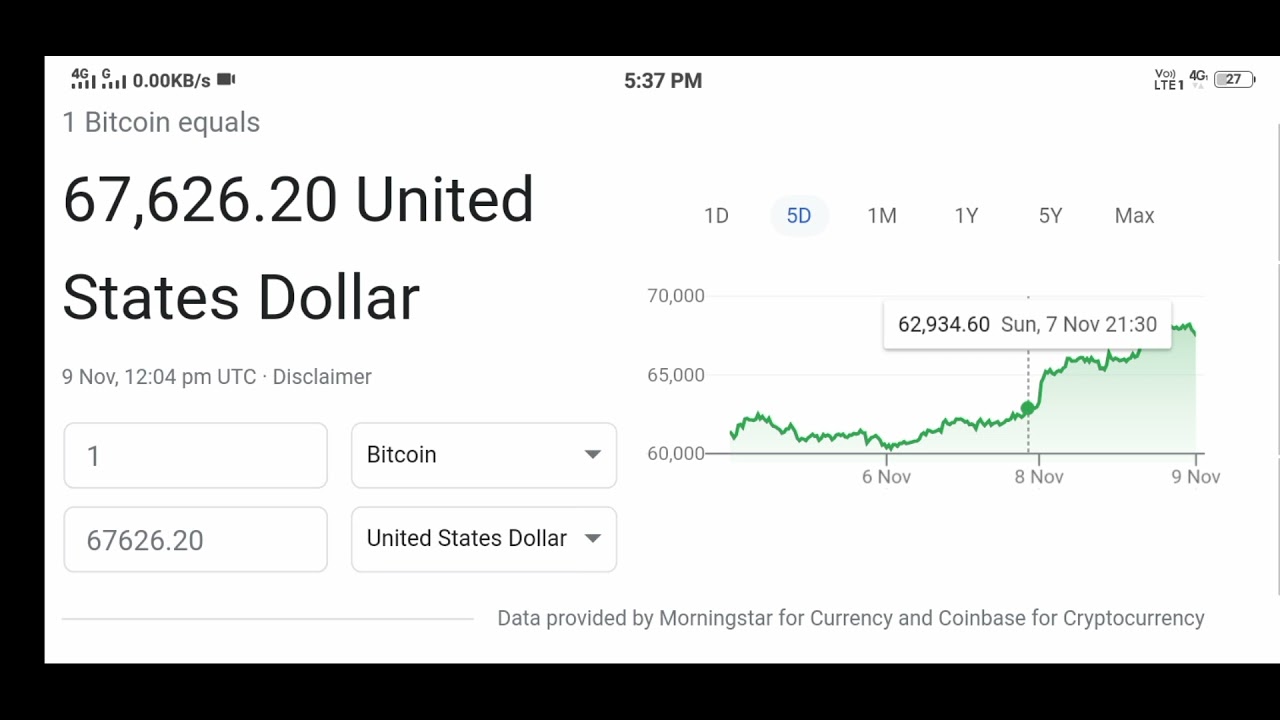Screenshot from a Bitcoin Tracking App on a Smartphone

The image captures a screenshot from a Bitcoin tracking app on a smartphone. Key details displayed in the image include:

- **Time and Date**: The screenshot was taken at 5:37 PM, with the data updated on November 9th at 12:04 PM UTC. The exact year is unspecified.
- **Phone Status**: The smartphone is connected to a 4G network with a battery level of 27%.
- **Bitcoin Value**: At the moment the screenshot was taken, the value of 1 Bitcoin is $67,626.20.
- **Data Providers**: The price data is sourced from Morningstar for currency and Coinbase for cryptocurrency.
- **Graph**: To the right, there is a chart tracking the recent fluctuations in Bitcoin value.

The detailed information reflects a snapshot of Bitcoin’s market value and the necessary technical conditions at the time of capture.